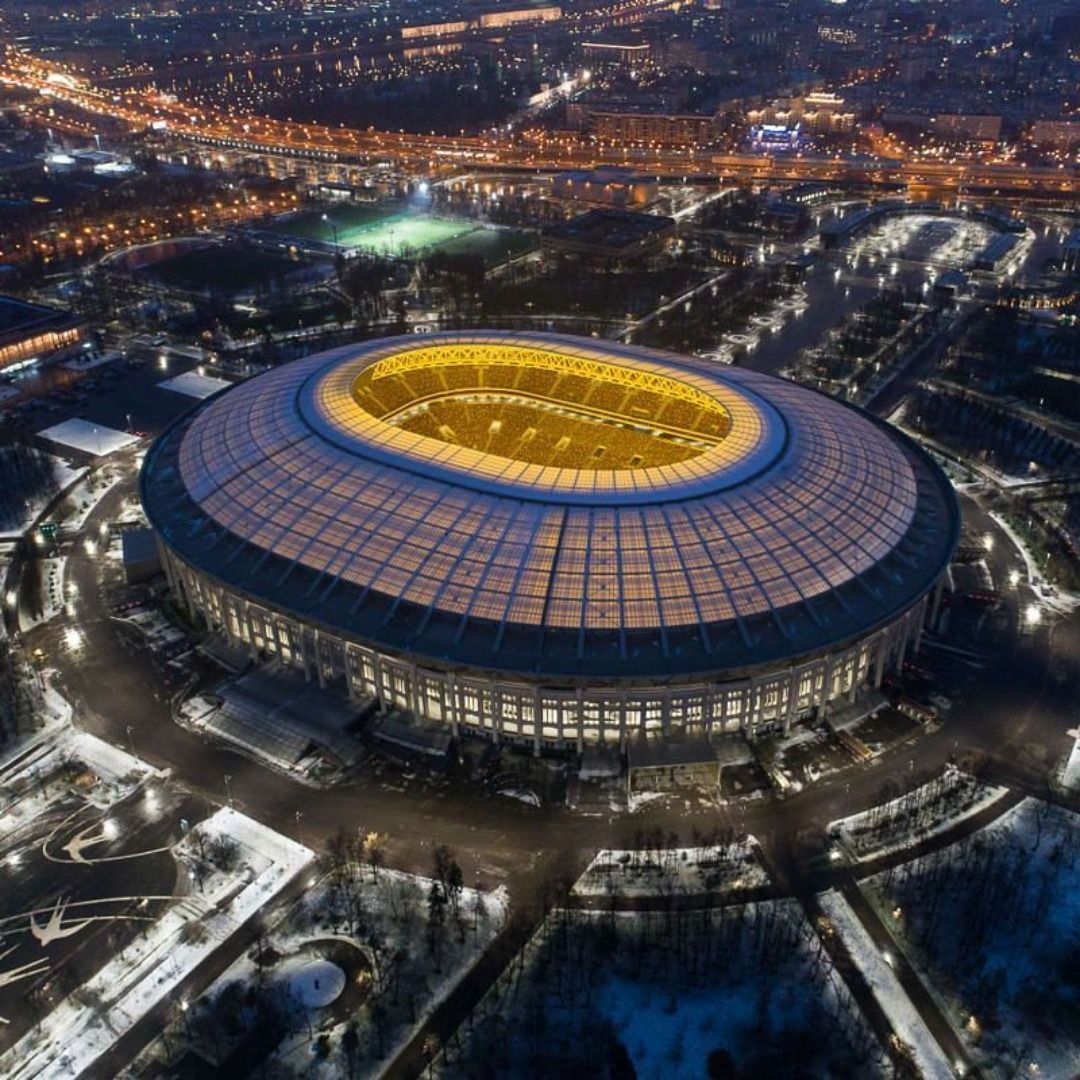This image captures a vibrant nighttime aerial view of an oval-shaped stadium in a major city, bustling with activity. The stadium, illuminated brilliantly, reveals numerous spectators inside as the roof is open, showcasing an actively used venue. Distinguished by its blue trusses and support beams, along with yellow seats that can be seen through the opening, the stadium gives off a vivid blue glow from the lighting on its dome and the yellow beam atop. The base of the stadium is whitish, enhanced with various windows emitting bright light.

Surrounding the stadium, a network of roads and winding streets leads to the venue, with a large circular road where cars are visibly moving. To the stadium's back left, there is a large tennis court, equally well-lit, adding to the urban landscape's complexity. Further behind the stadium, extensive city life is evident: multiple buildings and myriad lights stretch across the scene, and numerous cars travel along a large four-lane highway. This highway, alongside other smaller highways and roads intersecting the area, emphasizes the stadium's centrality in a very dynamic and densely built environment. The entire setting is framed by a snowy landscape with parcels of land sporting trees, completing the lively yet serene nighttime cityscape.